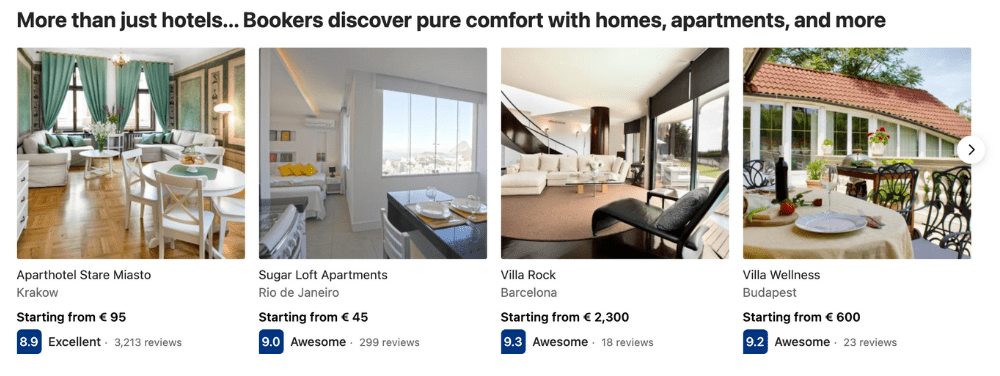Discover More Than Just Hotels: Immersive Stays for Every Lifestyle

Explore a world of comfort and convenience beyond traditional hotels with diverse home and apartment options available for booking. 

1. **Aparthotel Stare Miasto, Krakow**: Starting at 95 Lire, this establishment boasts an excellent rating of 8.9 from over 3,000 reviews. The spacious rooms feature elegant brown hardwood floors complemented by predominantly white furniture, including white tables and couches. Green tapestries adorn the wide-open windows, and large, beautiful pictures enhance the walls, creating a serene and elegant atmosphere.

2. **Sugarloaf Apartments, Rio de Janeiro**: With rates starting at 45 Lire, this stunning apartment has garnered an impressive rating of 9.0 from more than 299 reviews. The all-white setting exudes sophistication, illuminated by ample daylight streaming through the beautiful wide picture windows. The living space includes bright yellow pillows on the couches, adding a pop of color, and a kitchen countertop, making it a versatile and inviting environment.

3. **Villa Wellness, Budapest**: This luxurious villa, starting from 600 Lire, is rated an outstanding 9.2. The villa features an outdoor patio scene perfect for daytime relaxation or dining. The setup includes a wrought iron table set with food and chairs, under a red tile stucco roof of the white house adorned with large windows. Lush trees provide a picturesque backdrop, enhancing the villa's serene ambiance.

4. **Villa Rock, Barcelona**: With a starting price of $2,300 and an exceptional rating of 9.3, this villa offers a truly opulent experience. Highlighted by a spacious interior with white stone lighting, this property features a gigantic white couch set over a circular brown rug, comfortable lounge chairs, and an open patio. Outside, the patio hosts a table with a food setting, wrought iron chairs, and an exquisite view. This villa combines luxury with comfort, ideal for a premium stay. 

These meticulously selected properties showcase the varied and extraordinary accommodations available, ensuring every traveler can find their ideal home away from home.